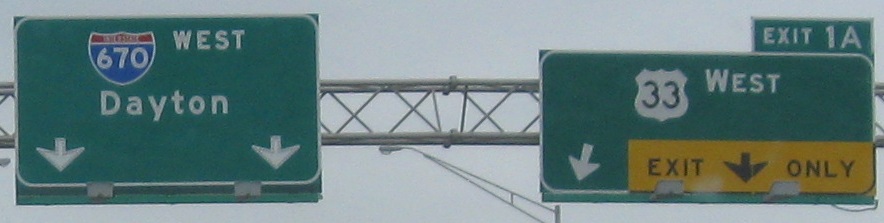This is a color photograph showcasing two prominent green highway signs positioned side by side, both securely attached to a wide, horizontal metallic framework. Connecting these signs are two horizontal metal bands, reinforced by an intersecting X-shaped support structure.

On the left sign, "Dayton" is clearly written in white uppercase letters against the green background. Positioned at the top edge of this sign is the word "West" in white, indicating the direction. Below "West," there is an Interstate shield emblem in blue and red, marked with the number "670." Two white arrows point downward beneath "Dayton," guiding drivers toward the appropriate lanes.

The right sign features the number "33" in bold white, followed by "West." Below this, there is also a downward-pointing white arrow. Attached to this sign is a smaller, vibrant yellow rectangle with black lettering that reads "Exit Only," accompanied by another downward arrow. Additionally, a compact green sign is located towards the upper right corner of the larger sign, displaying "Exit 1A" in white letters. This smaller sign is supported by a diagonal line that adds to the intricate web of metallic reinforcements.

The detailed array of directional cues and exit information provided by these signs serves to guide the drivers accurately and ensure smooth navigation on the highway.